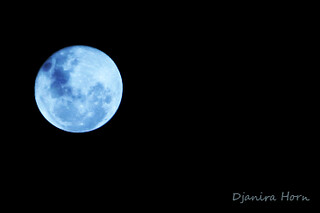This is a simple yet striking photograph capturing a landscape layout. The photograph features a solid black background, dominated by a detailed image of the moon on the left third, centered vertically. The moon itself emits a whitish-blue hue, illuminating its surface details with varied shades of white, blue, and almost black, highlighting its craters and elevations. The right side of the moon appears slightly lighter than the left side, adding depth to the celestial depiction. In the lower right-hand corner, the photographer's name, D. Janera Horn, is elegantly inscribed in cursive white text, affirming the creator's identity. The entire scene is minimal yet profound, focusing solely on the moon against the absolute darkness.